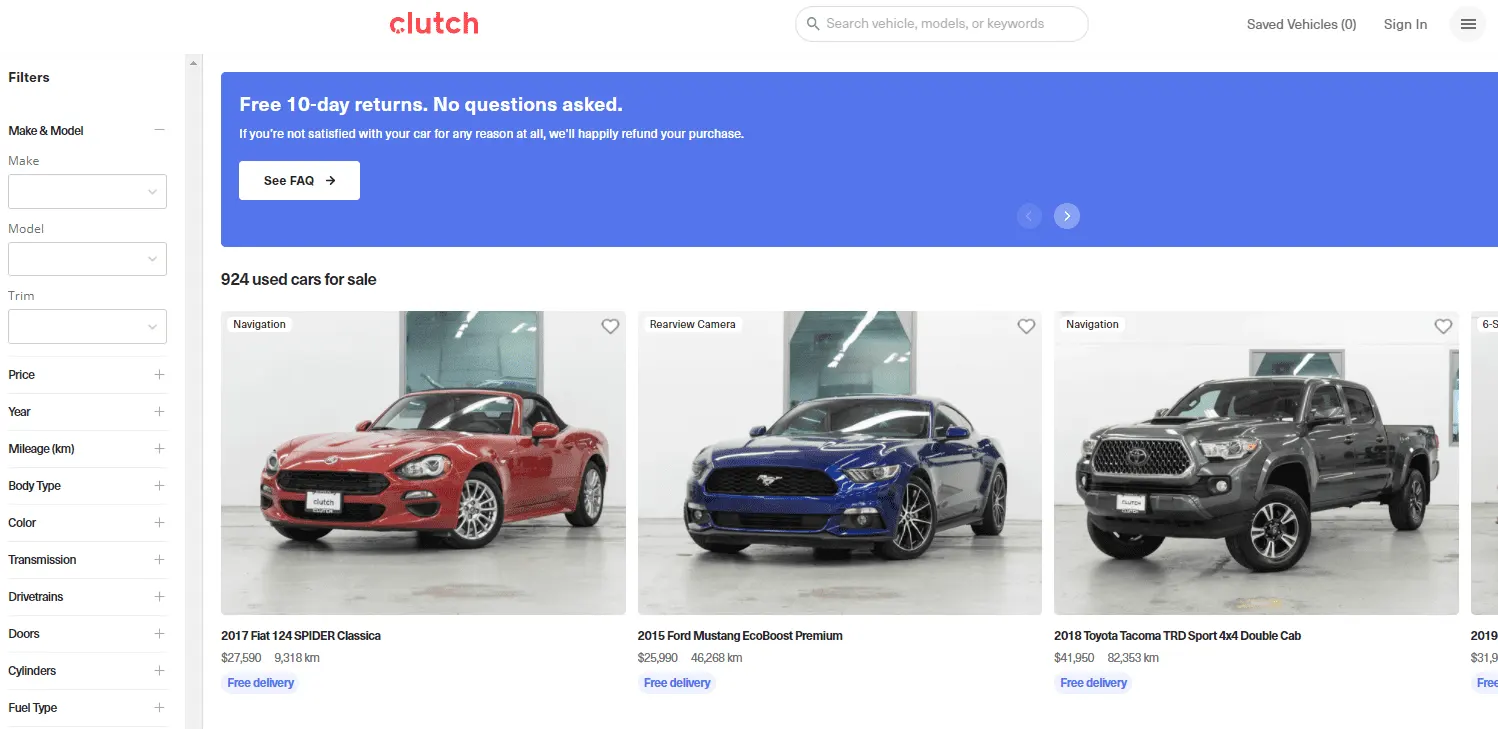Here's a cleaned-up and detailed caption for the described image:

"Three vehicles are showcased: a striking red sports car, a sleek blue sports car, and a robust black pickup truck. Specifically, they are:

1. A 2017 Fiat 124 Spider priced at $27,000 with an odometer reading of 9,000 kilometers. It includes free delivery.
2. A 2015 Ford Mustang EcoBoost Premium available for $25,000, having traveled 46,000 kilometers, also with free delivery.
3. A 2018 Toyota Tacoma TRD Sport 4x4 Double Cab listed at $41,950 with 82,363 kilometers on the clock, featuring clutch-free operation and free delivery.

All vehicles come with a hassle-free 10-day return policy. If you're not satisfied with your purchase for any reason, we offer a no-questions-asked refund. Explore our collection of 924 used cars for sale using various filters such as make, model, trim, price, year, mileage, body type, color, transmission, drivetrain, doors, cylinders, and fuel type. You can search for vehicle models or keywords, and save your favorite vehicles. Sign-in available for a personalized experience."